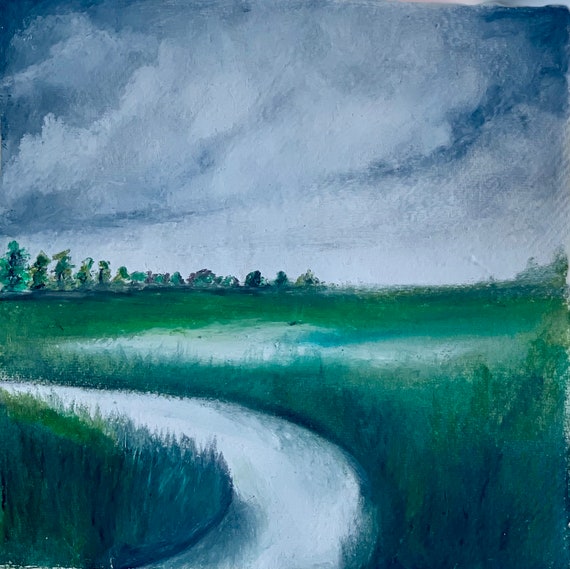This oil painting depicts a dreary outdoor scene dominated by a meandering river that begins in the center bottom of the canvas and curves gently to the right before veering off to the left. The river's blue waters contrast sharply against splotches of green grass on either side, which appear bluish-gray in some areas due to abstract artistic touches. In the lower left corner, a notable patch of grass stands out before it is enveloped by the river. The grassy field surrounding the river varies in color, showing hints of white in the middle, hinting at a swampy area. Moving beyond the field, along the horizon, a line of trees can be observed, becoming denser and larger towards the left. Above this tranquil yet somber landscape, the sky is painted in dark, moody hues of blue, filled with heavy clouds, adding to the overall dreary atmosphere of the scene.